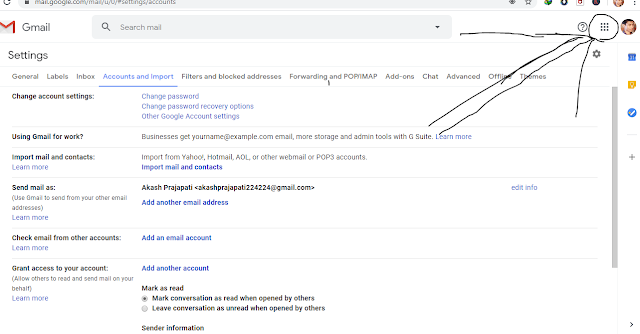The image is a screenshot of an email settings page within Gmail, accessed through a web browser. The background is a stark white, blending seamlessly into the browser's white interface. At the top of the screen, the URL displayed is "mail.google.com," indicating that the user is on the Gmail website. Directly below the URL bar is a prominent Gmail search bar designed for searching emails. 

The central focus of the screenshot appears to be the "Accounts and Import" tab within the Gmail settings, the fourth tab among others such as General, Labels, and Themes, highlighted in blue and underlined. Within this tab, different sections are available, including "Change account settings," "Using Gmail for work," and "Import mail and contacts," among others.

In the upper right corner of the screen, next to the user's profile picture, is a grid icon featuring nine dots arranged in a 3x3 grid. This icon is circled and annotated with a double-lined arrow pointing towards it, likely drawn with a pen tool. The arrow, composed of two parallel lines with a single-lined V-shaped head, emphasizes the grid icon, probably to highlight its importance or function.

This annotation suggests that the image was modified to draw specific attention to the grid icon, possibly to indicate its use or to instruct someone to click on it.